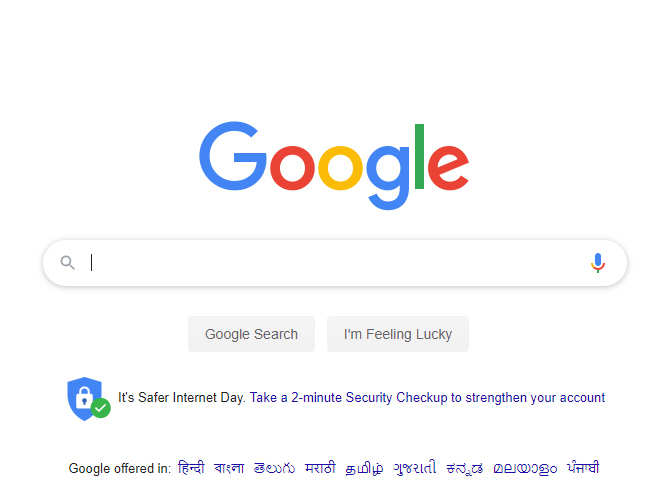The image features the Google search bar prominently centered. The word "Google" is displayed in its signature multi-colored letters: both 'G's are blue, the left 'O' is red, the right 'O' is yellow, the 'L' is green, and the 'E' is red. The search bar itself has a blinking cursor in the prompt area. On the left side of the search bar, there is a gray magnifying glass icon, while on the right side, there is a small microphone symbol, indicating voice search functionality. 

Below the search bar are two gray buttons. The button on the left reads "Google Search," and the button on the right reads "I'm Feeling Lucky." Beneath these buttons, there's a notification featuring a blue shield with a white lock icon and a green circle with a white checkmark. The notification text reads, "It's Safer Internet Day. Take a two-minute security checkup to strengthen your account."

Further down, it says, "Google offered in," followed by some text written in a script resembling either Hindi or Thai. The background of the screen is white, and the search bar is outlined with a subtle gray shadow to make it stand out from the page.